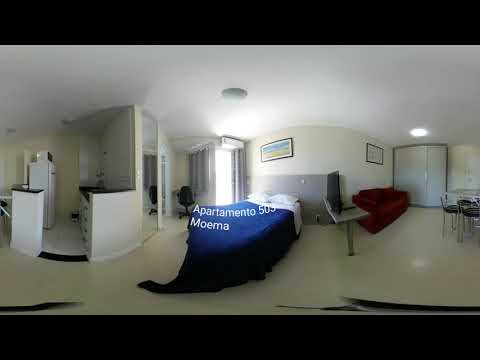This is a panoramic photograph of a sleek and modern studio apartment. The left side of the image features a small, open-concept kitchen with white cabinets, a black countertop, a two-burner stove with an oven underneath, and a white fridge. In the center of the apartment is a bed with a blue comforter, white sheets, and pillows, adorned with white letters spelling "Apartamento 503" and "MOMA." A black or cranberry-colored sofa sits to the right of the bed, near a white closet or cabinet. Adjacent to the sofa is a desk with a computer screen. A small round kitchen table with chairs is partially cut off on the far right side of the panoramic view. The apartment has white or off-white walls and ceiling. The furnishings are minimal, including some bland pictures on the walls, and the overall space appears slightly distorted due to the panoramic stitching.